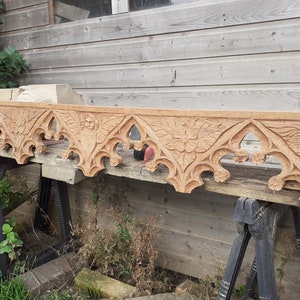The image depicts a close-up view of an unpainted, intricately carved wooden architectural piece with a distinct Victorian and gothic style, resting against the light whitish-gray wooden siding of an outdoor structure, likely a barn or garage. This decorative element, resembling what one might place at the edge of a house or beneath a roof, features a series of interlinked triangles adorned with elaborate carvings of leaves, flowers, and angels. The piece is supported by two black plastic sawhorses, sitting on a wooden bench or board. The ground below shows a mix of green leafy plants, dried brown vegetation, and several gray cinder blocks scattered across the area. In the background, there's a hint of windows cut off at the top of the picture, and the scene appears set for further work, possibly painting or installation.